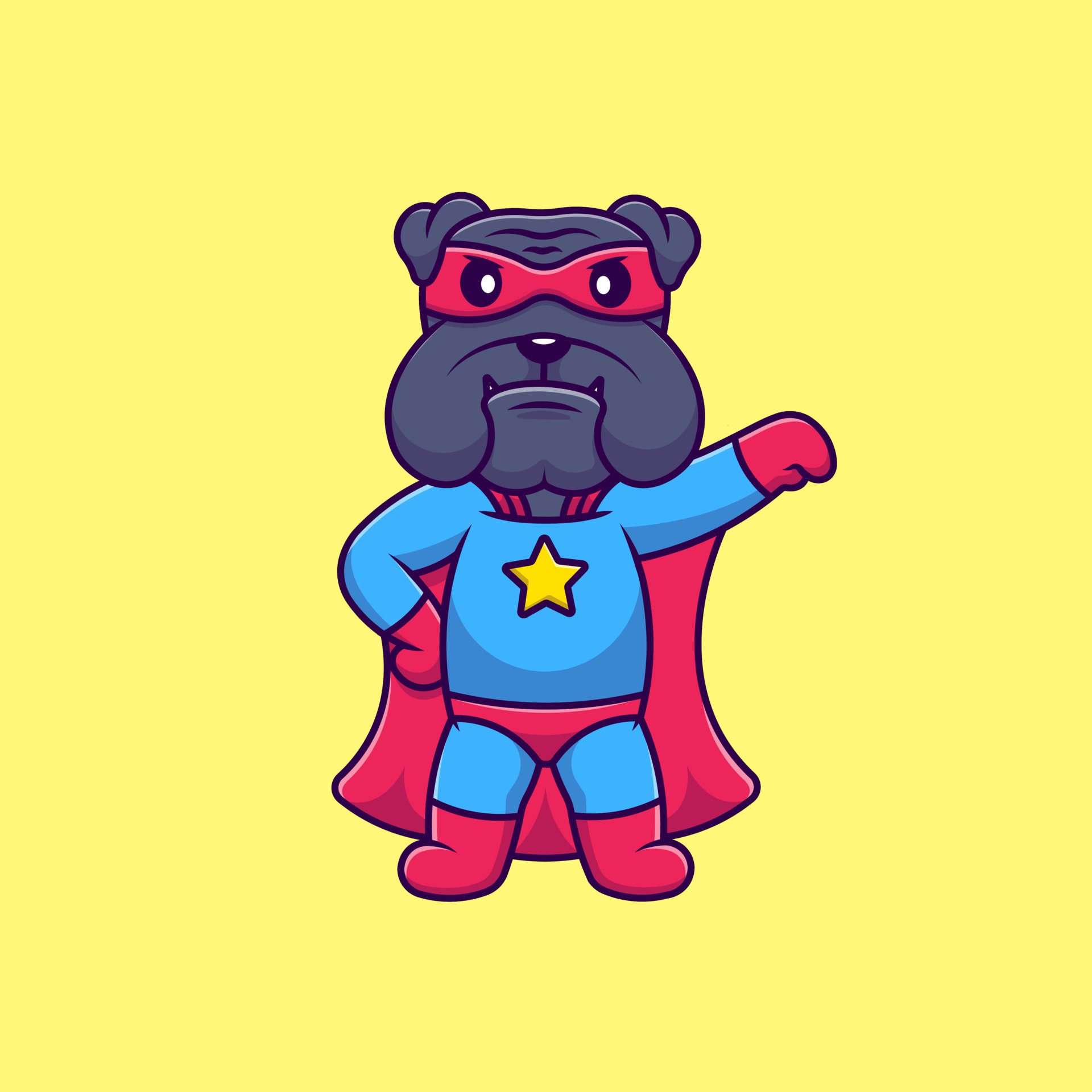This is a detailed illustration of a cartoon gray bulldog dressed as a superhero, set against a bright yellow background. The bulldog, with dark gray fur and two floppy ears almost covering its eyes, faces directly forward. The dog dons a classic Superman-style costume, consisting of blue tights, a long-sleeved blue shirt with a prominent gold star emblazoned in the center, and a pair of red briefs. His red superhero attire extends to accessories, including a red mask tied around his head, matching red mittens, and red boots. Standing anthropomorphically on his hind legs, the bulldog strikes a heroic pose: his left paw is raised and extended straight from the shoulder as if ready to take flight, while his right paw rests confidently on his hip. His large jowls, small black nose, and sharp canine teeth are distinctly bulldog-like, enhancing the endearing yet formidable superhero persona.